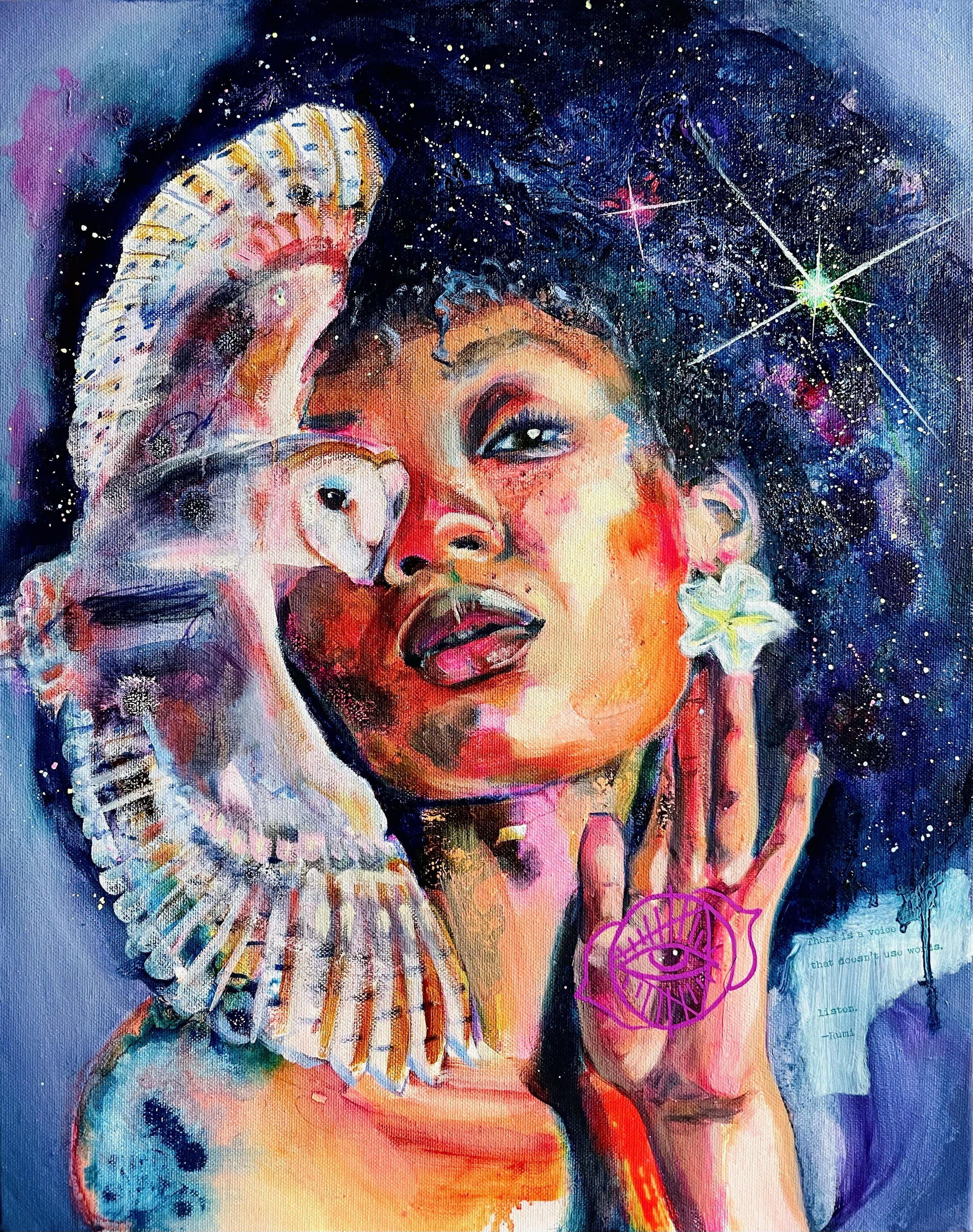The image is a vibrant and abstract painting of an African American woman, set against the backdrop of a colorful galaxy. The woman, depicted with cartoonish features, has a brown complexion, purple lips, and red rouge on her cheeks. Her black hair stands straight up, resembling the vast universe with specks of stars and clouds in bluish hues. She holds her left hand up to her face, adorned with a blue flower earring and a tattoo of an eye with fins on her palm. A majestic white owl with wings tipped in darker purples and abstract colors appears to be crashing into her right eye, covering that side of her face and body. The background bursts with blues, purples, and pinks, contributing to the cosmic feel of the piece. The woman’s neck displays a mix of purple, brown, and yellow hues. Toward the bottom right-hand corner, there is a cutout of some writing that reads, “There is a voice that doesn't use words, listen, woomy.” The image is rich in symbology, blending elements of protest art and children's abstract paintings, creating an evocative and powerful visual narrative.